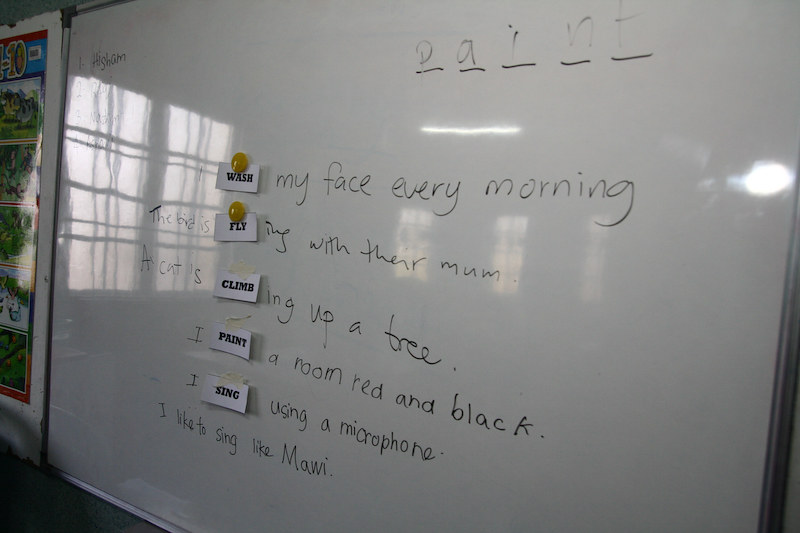In this classroom scene, a dry erase whiteboard is prominently displayed. At the top right corner, the word "PAINT" is written with each letter underlined. The board features a teaching aid where students appear to be learning English sentences through a matching exercise. Five key verbs—'wash,' 'fly,' 'climb,' 'paint,' and 'sing'—are printed on separate pieces of paper and affixed to the board with magnets. Each verb corresponds to a sentence written in black marker next to it. The sentences read: "I wash my face every morning," "The bird is flying with their mom," "A cat is climbing up the tree," "I paint a room red and black," and "I sing using a microphone." On the left side of the board, there's a poster, contributing to the classroom's learning environment.